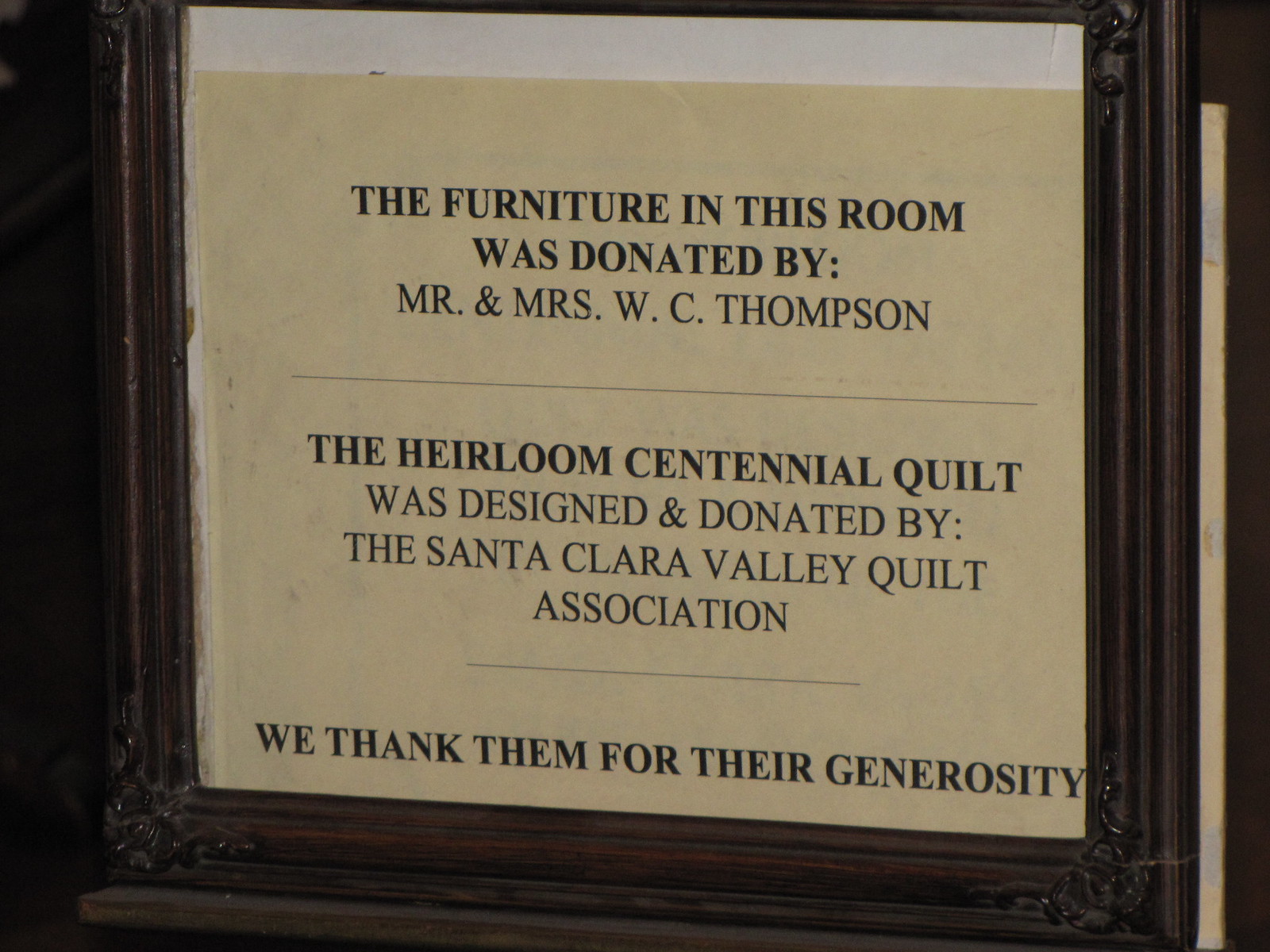The image is a color photograph of a sign enclosed in a dark mahogany wooden frame. The inside of the frame features a cream-colored background with black writing. The text on the sign reads: "The furniture in this room was donated by Mr. and Mrs. W.C. Thompson. The Heirloom Centennial Quilt was designed and donated by the Santa Clara Valley Quilt Association. We thank them for their generosity." Certain parts of the text, such as the donors' names, the name of the quilt, and the expression of gratitude, are emphasized in bold.